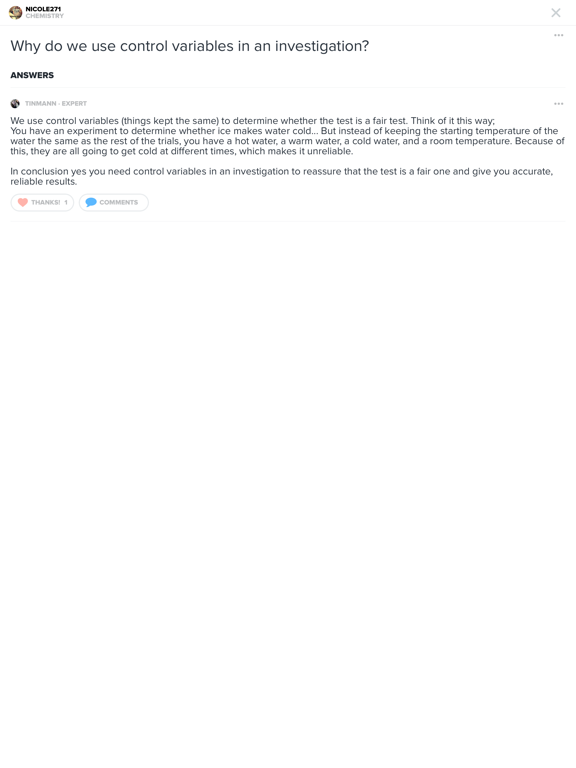The image features a small, concise text snippet on the topic of control variables in scientific investigations. At the top left, the text reads "NICOLE271 CHEMISTRY" in bold letters, clearly identifying the subject of the discussion. Below this heading is a small icon depicting a person, followed by the text in gray, stating "seems to be the hit thing."

The main content is a detailed explanation provided by "TinManExpert." The explanation discusses the importance of using control variables in scientific investigations to ensure fair and reliable results. It explains, for instance, why maintaining consistent starting conditions, such as the initial temperature of water in an experiment involving ice, is crucial. Without these consistent starting conditions, different variables such as hot water, warm water, cold water, and room temperature water would influence the results, leading to unreliable conclusions.

In summary, the text emphasizes that control variables are essential in conducting fair and accurate scientific tests. Following the explanation, there are interactive icons- a heart labeled "thanks" and a blue thought cloud labeled "comments," inviting users to engage with the content. The caption ends with a brief, encouraging reminder: "Yeah, use your variables."